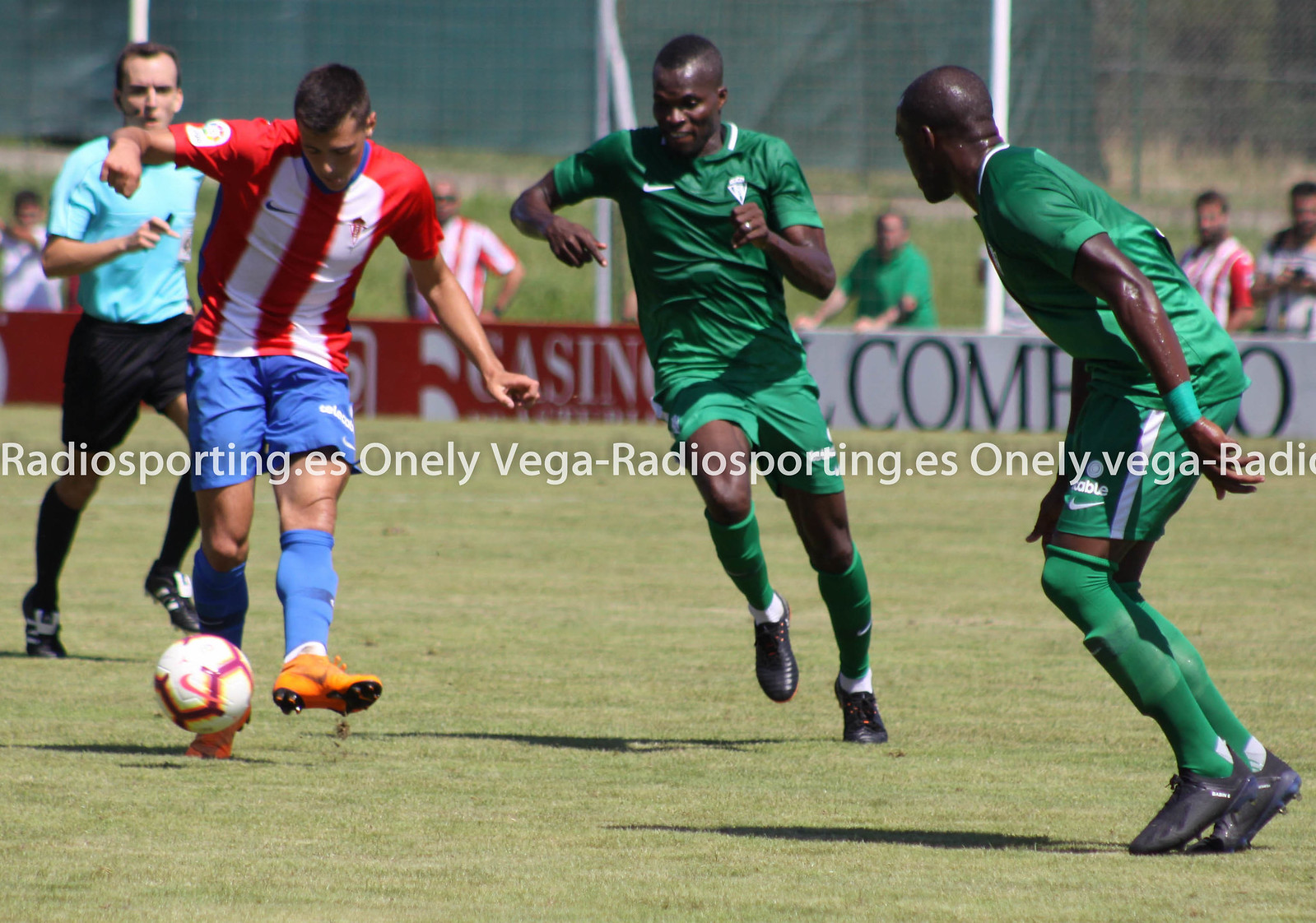In this vibrant and detailed action shot of a live soccer game, three players and a referee are captured mid-play on a lush green grass field. On the left, a player in a red and white striped jersey, blue shorts, and blue socks is seen controlling a red and white soccer ball. He is intensely focused, looking down as he is about to kick the ball. To his right, two African men in matching green uniforms, including green jerseys, shorts, and knee socks, are in motion, possibly closing in to challenge for the ball. One of them is wearing bright orange cleats, emphasizing the dynamic movement with dirt visibly kicked up from the field. Behind them, a referee wearing a light blue shirt and black shorts, equipped with an earpiece and microphone, attentively observes the action. In the background, a viewing area with banner ads and spectators can be seen, further highlighting the realism and energy of the game.